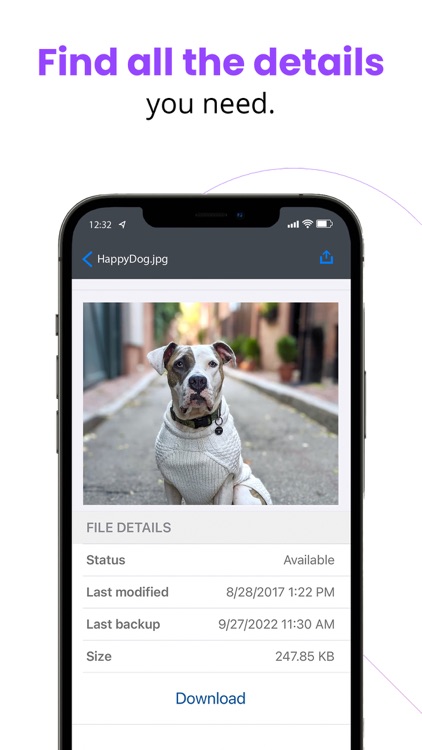The image depicts a screenshot of a cellphone interface, specifically showcasing a photo details screen. At the top, in bold purple letters, the text reads "Find All the Details" with the supporting text "you need" in regular black font directly beneath it. 

Central to the screenshot is an image of an iPhone, recognizable by its distinct volume buttons, power button, camera, and speaker layout. The device's status bar at the top left corner displays the time as 12:32, and a location icon is also visible. On the right side of the status bar, there are icons indicating cellular service strength, WiFi connectivity, and battery level. The top section of the screen is shaded gray, featuring a blue arrow on the left for navigation, the file name "happydog.jpg" in the center, and an icon on the right to save or share the photo.

The primary focus of the image is a photo of a dog. The dog has predominantly white fur with distinctive brown and black markings around its left eye. Additionally, there is a brown patch on the right side of its face, away from the eye. The dog is donned in a knit white sweater.

Below the photo, detailed file information is provided. It includes:
- File Details
- Status: Available
- Last Modified: 8-28-2017, 1:22 PM
- Last Backup: 9-27-2022, 11:30 AM
- Size: 247.85 KB

At the very bottom of the screen, a blue "Download" button is situated.